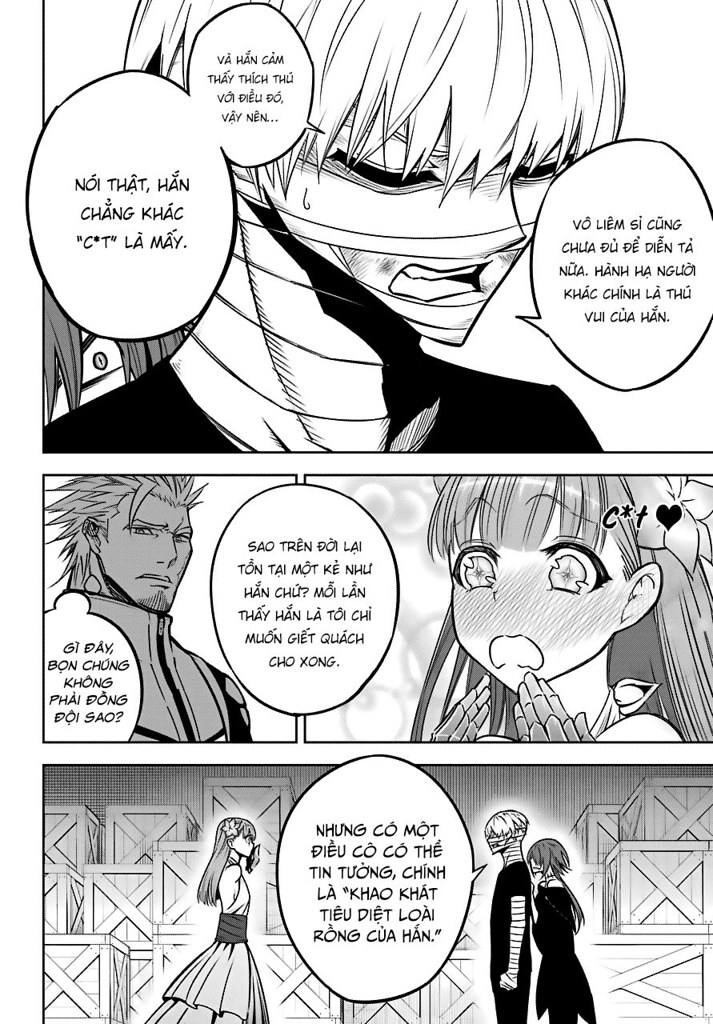This black-and-white graphical novel or comic book is composed of three horizontal panels, each rich in detail and storytelling. The uppermost panel features an extreme close-up of a man with long blonde hair draping over his eyes in an Asian or anime-inspired style. His face and body are partially obscured by bandage-like wrappings, giving him a mummy-esque appearance. Vertical lines dominate the background as three speech bubbles emanate from him, text written in what appears to be either Vietnamese or Cambodian.

In the middle panel, the scene splits into two sections. On the left stands a burly man with spiky blonde hair, partially visible from the chest up and wearing a high-collared jacket that accentuates his powerful presence. To his right is a traditional anime-style girl, distinguished by her long hair, wide eyes, and gloved hands raised to her mouth in an expression of fear or shock. Both characters are engaged in dialogue with foreign language speech bubbles.

The bottom panel brings all three characters together. On the left is the anime-style girl dressed in a long gown, engaging with the man from the top panel on her right. He is now dressed in a black t-shirt and black pants, with bandage-like stripes on his arms and face. Next to him stands another woman, also in a black dress, with long dark hair and her hands resting gently on his back. The background hints at a warehouse setting with wooden boxes stacked behind them. The speech bubbles suggest a conversation, again written in the foreign language consistent with the previous panels.